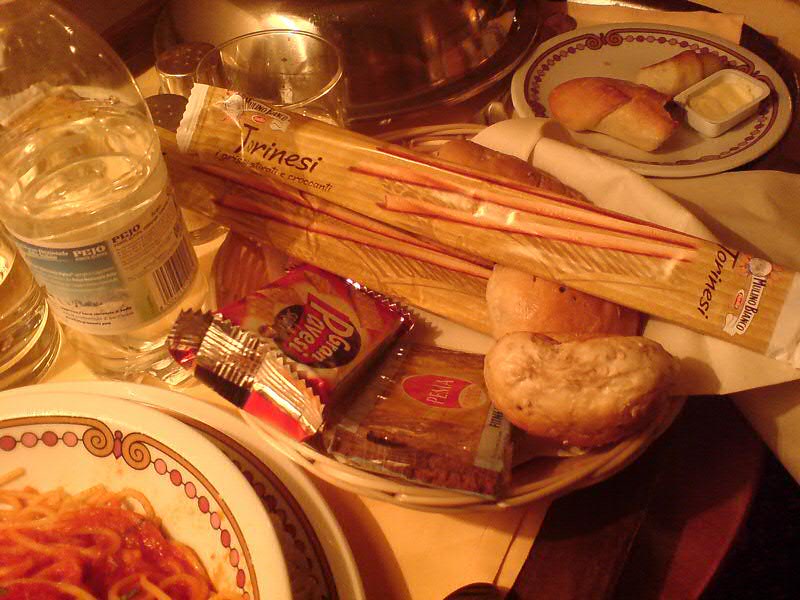This photograph, likely taken at an Italian restaurant or as room service in a hotel, showcases a beautifully arranged tray of food on a customer's table. In the bottom left corner, a retro-patterned bowl with pink, red, and yellow dots and a gold fringe border holds spaghetti topped with red sauce. Next to it, a wicker basket rests in the center, containing an assortment of packaged breadsticks, rolls, and crackers, labeled Gran Pavese, Pima, and Turinesi. An accompanying bottle of water stands beside it. Toward the upper right, a smaller plate features rolls, one partially eaten, alongside a small tub of butter. A silver-covered dish is positioned further up in the image, with salt and pepper shakers standing slightly to its left. A glass is also visible near the central basket, contributing to the impression that the meal is in progress. The assortment of dishes, complete with a napkin beneath the bread basket, evokes a sense of a hearty and partially consumed meal set in a cozy dining atmosphere.